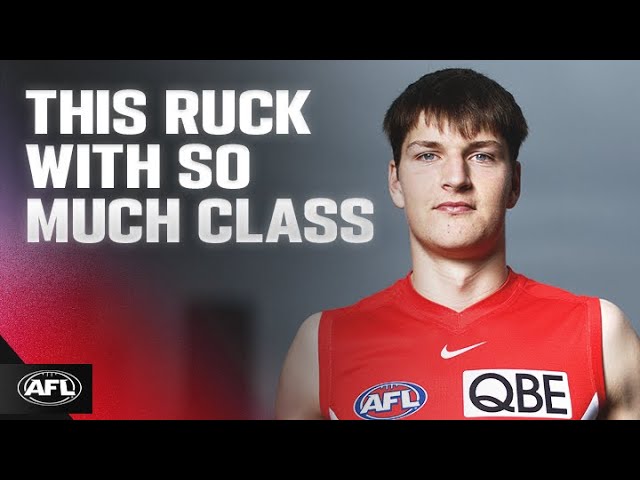In this image, a young man with short, dark hair and a serious expression is positioned on the right side, gazing into the camera. His light eyes and prominent Adam's apple accentuate his features. He is wearing a high v-neck, sleeveless red jersey adorned with several logos: a white Nike emblem, a white, blue, and red AFL logo, and a rectangular black and white QBE patch. The AFL logo appears twice in the image: once on his jersey and again in a smaller black and white version in the bottom left corner. On the left side of the picture, large white text reads, "this ruck with so much class." The backdrop is a mix of gray, fading into pink and purple hues that are out of focus, contributing to the image's depth. The image is framed by two thick black stripes at the top and bottom, adding a sense of structure to the composition.